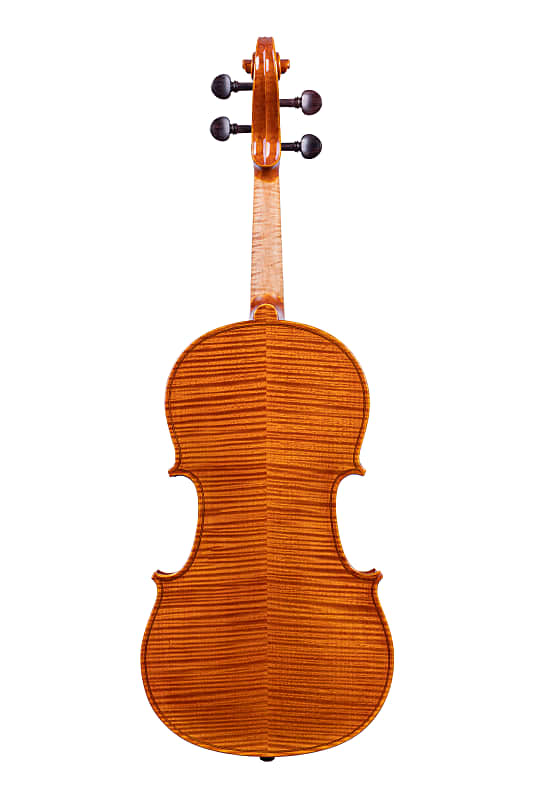The image showcases a beautifully crafted violin, rendered in a detailed, almost hand-drawn style. The instrument, displayed against a white background, reveals the back side of the violin, distinguished by its rich dark red color with intricate wood grain patterns and stripes. This violin is equipped with four black tuning pegs—two on each side of the headstock. The neck of the violin exhibits a smooth transition from the darker wood of the body to a lighter shade, emphasizing the quality craftsmanship. At the bottom lies a small black endpin, designed to protect the instrument when placed on the ground. The bronze-to-brown hues at both the top and bottom add a touch of elegance, further enhancing the violin's professional and classical appearance. This exquisite violin likely belongs in a symphony, indicative of an instrument that a musician would invest significantly in.